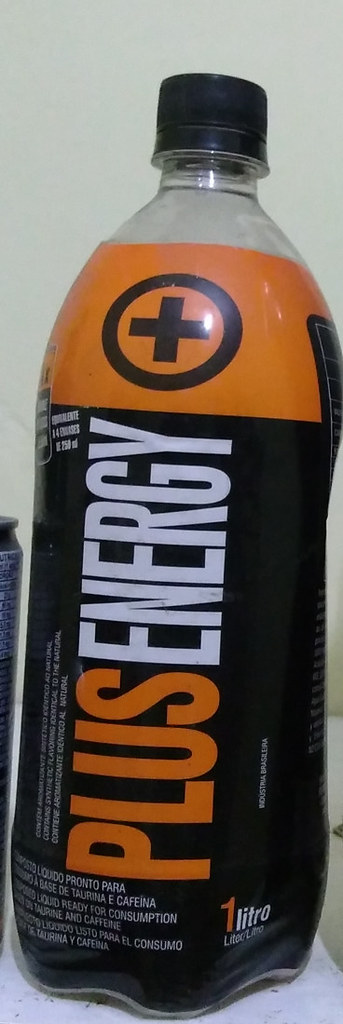This close-up photograph features a bottle, likely containing an energy drink, prominently displayed against a minimalistic white surface. The bottle's design is distinct, with a robust and thick body tapering into a narrower top, capped with a black plastic lid. Its base is scalloped, reminiscent of the bottom of a liter of soda, adding texture to its silhouette. The label is striking, starting with an orange band at the top that encloses a black plus symbol within a circle. Running vertically down the center, orange text spells out "Plus" followed by "Energy" in white letters set against a black background. Below the main branding, smaller text in white provides additional product information, contributing to the overall sleek and energetic aesthetic of the bottle.